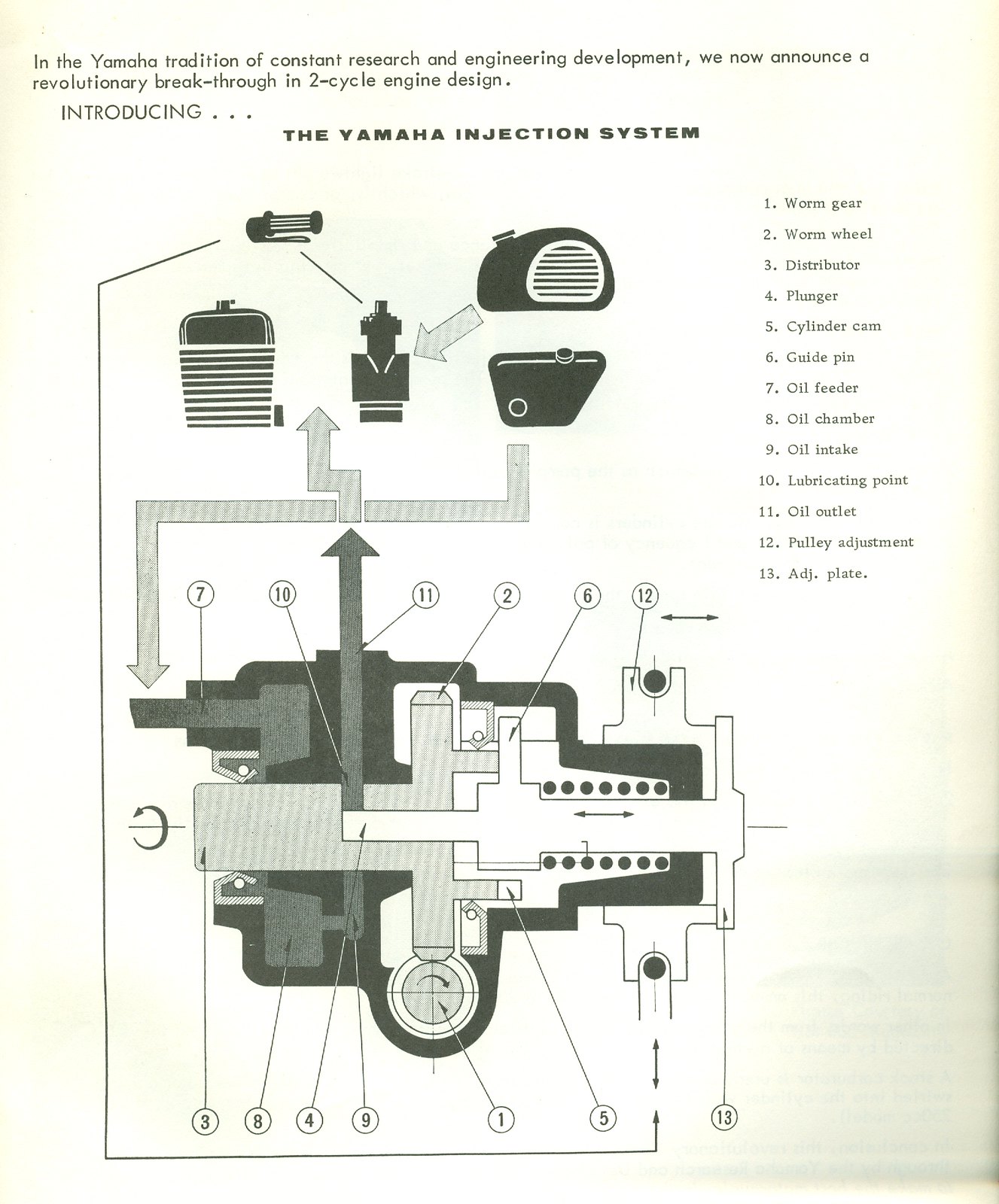The image features a detailed, grayscale blueprint of the Yamaha Injection System, emphasizing Yamaha's tradition of constant research and engineering development. At the top, the text reads, “In the Yamaha tradition of constant research and engineering development, we now announce a revolutionary breakthrough in two-cycle engine design—introducing the Yamaha Injection System.” The central diagram showcases various components of this injection system, with 13 parts meticulously labeled: Worm Gear, Worm Wheel, Distributor, Plunger, Cylinder Cam, Guide Pin, Oil Feeder, Oil Chamber, Oil Intake, Lubricating Point, Oil Outlet, Pulley Adjustment, and Adjusted Plate. Each part is connected to numbered points, showing its specific location and role within the system. Other visual elements include an oval-shaped machine with a grill, a display attached to a person with a rolling handle, and a shampoo-bottle-like object with dashed lines. Arrows throughout the blueprint provide a comprehensive guide to the assembly and function of the system.